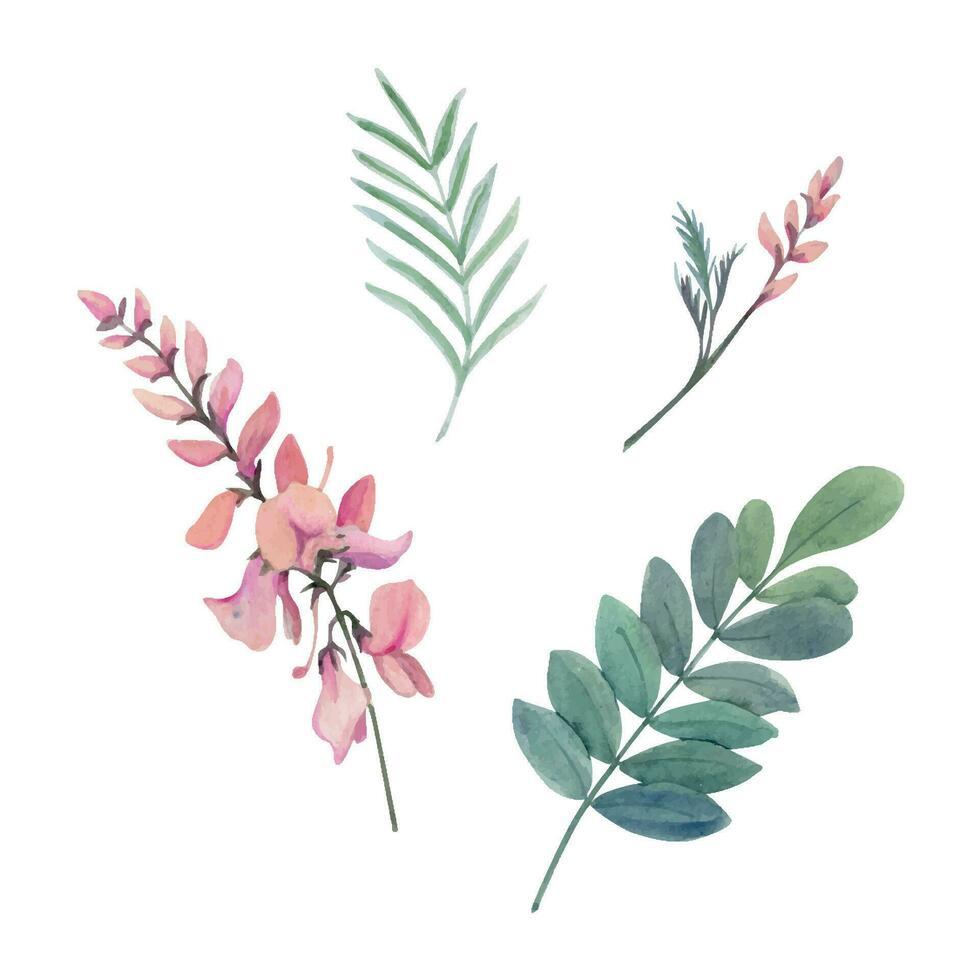The image features a highly detailed, textbook-like botanical illustration set against a crisp, white background, displaying four distinct plant elements. In the top-left corner, there is a depiction of a light green fern with a single central stem and six long, skinny leaves branching off symmetrically on each side, one large leaf in the middle. To the right of the fern is a stem adorned with pink flowers, characterized by buds at its tip and three foamy-looking, spiked leaves on the left. The bottom-left segment is a close-up of the same pink flower, highlighting its vibrant, darker pink center and lighter pink outer petals, with multiple buds at various stages of blooming. On the bottom right of the image, another stem showcases several green leaves, including a prominent rounded leaf at the top, flanked by smaller leaves on either side. The artistic rendering emphasizes the natural beauty and unique characteristics of each plant part with intricate detail.